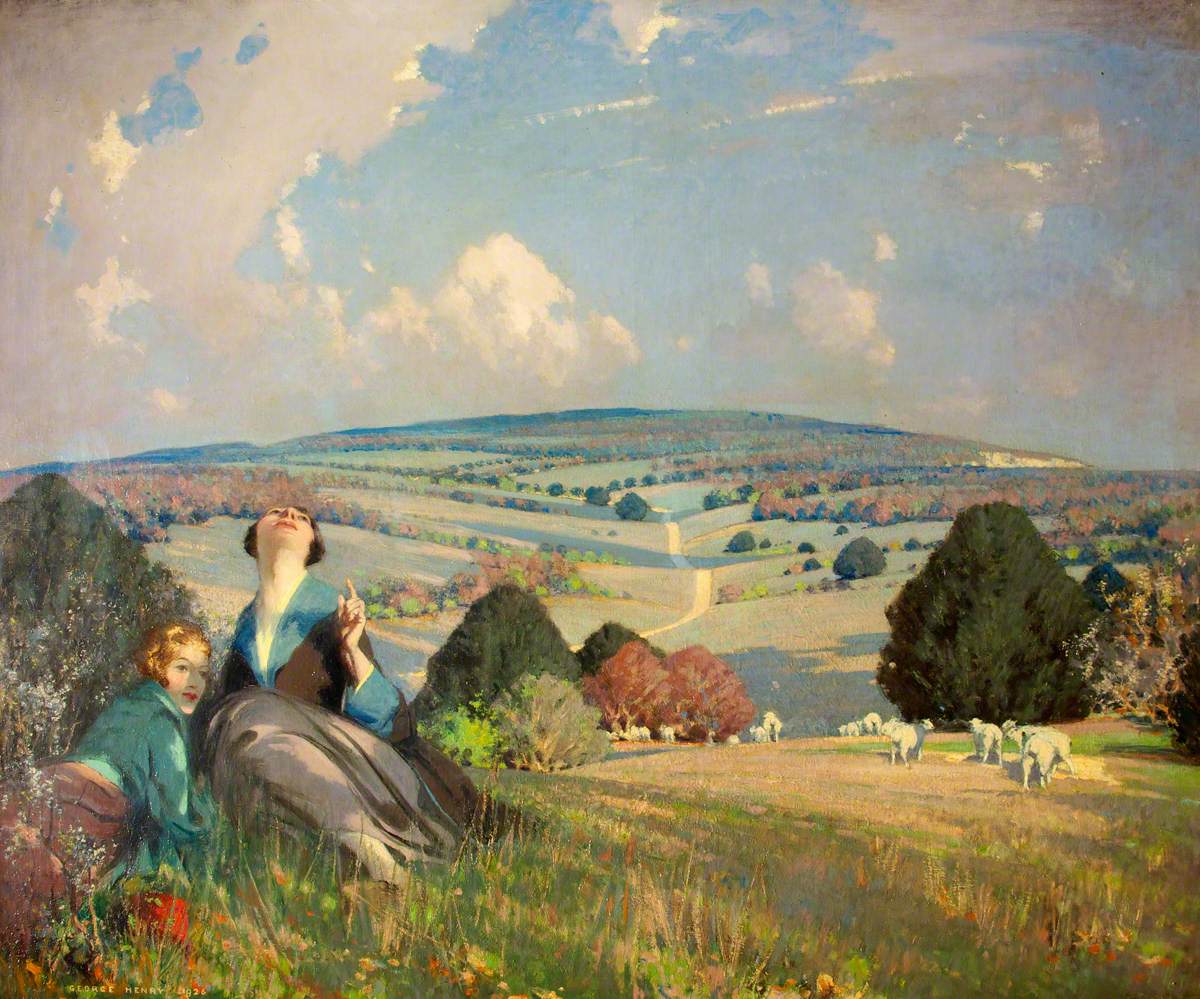This painting, likely from the late 19th or early 20th century, captures a serene autumnal landscape of rolling hills beneath an expansive sky filled with billowy white clouds. Central to the scene are two women in old-fashioned attire of long skirts and blouses. They sit amidst tall grass adorned with multicolored wildflowers on the left side of the composition. One woman points skyward with her left hand, her gaze following her finger toward the heavens, while the other reclines, looking contemplatively off toward the viewer's perspective. The foreground is dotted with grazing sheep and interspersed with trees in varying autumnal hues—some still green, others brown or red, signaling the change of seasons. A winding road snakes through the valley, framed by bushy trees, adding depth and leading the eye through the tranquil countryside. The detailed depiction of the landscape and the women’s interaction with their surroundings evoke a sense of peaceful admiration and timeless beauty.